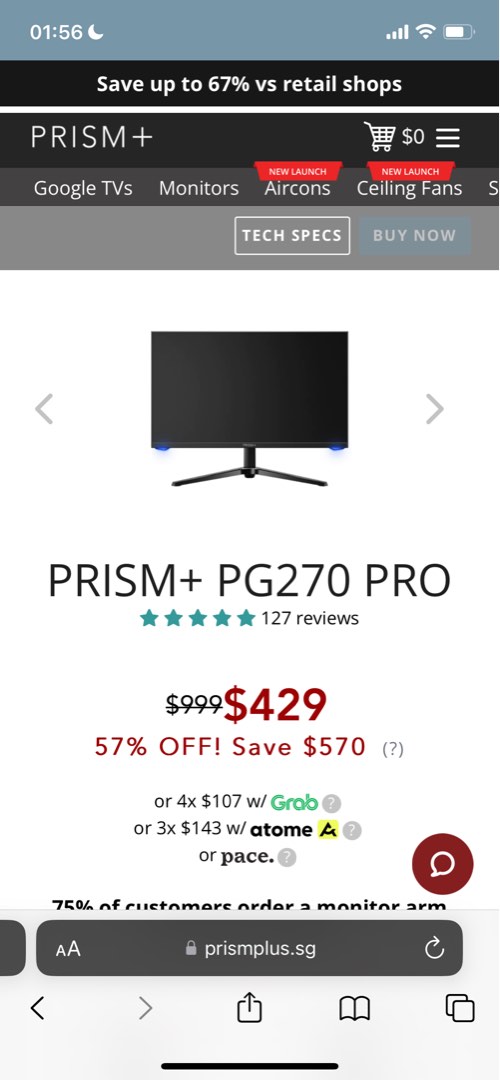This image depicts a mobile device displaying the Prism+ website, which specializes in selling technology products. The device is held vertically, and at the top of the screen, a blue status bar shows the time as 1:56, along with indicators for internet connection, service, and battery life, which is approximately 75% charged.

Below the status bar, there's a prominent black banner with white text declaring "Save 67% versus retail shops." Underneath this, a gray header bar displays the Prism+ logo on the left and an empty shopping cart icon on the right, indicating a zero-dollar balance.

Further down, a navigation bar provides tabs for various categories of products sold on the site, including Google TVs, monitors, air conditioners, and ceiling fans. Below these tabs, actionable buttons labeled "Tech Specs" and "Buy Now" are prominently displayed.

The main product being viewed is highlighted with a significant discount, marked in red text: "57% off, Save $570" reducing the price from $999 to $429. Additionally, there are payment options available, allowing the customer to pay in installments of four times $107 or three times $143.